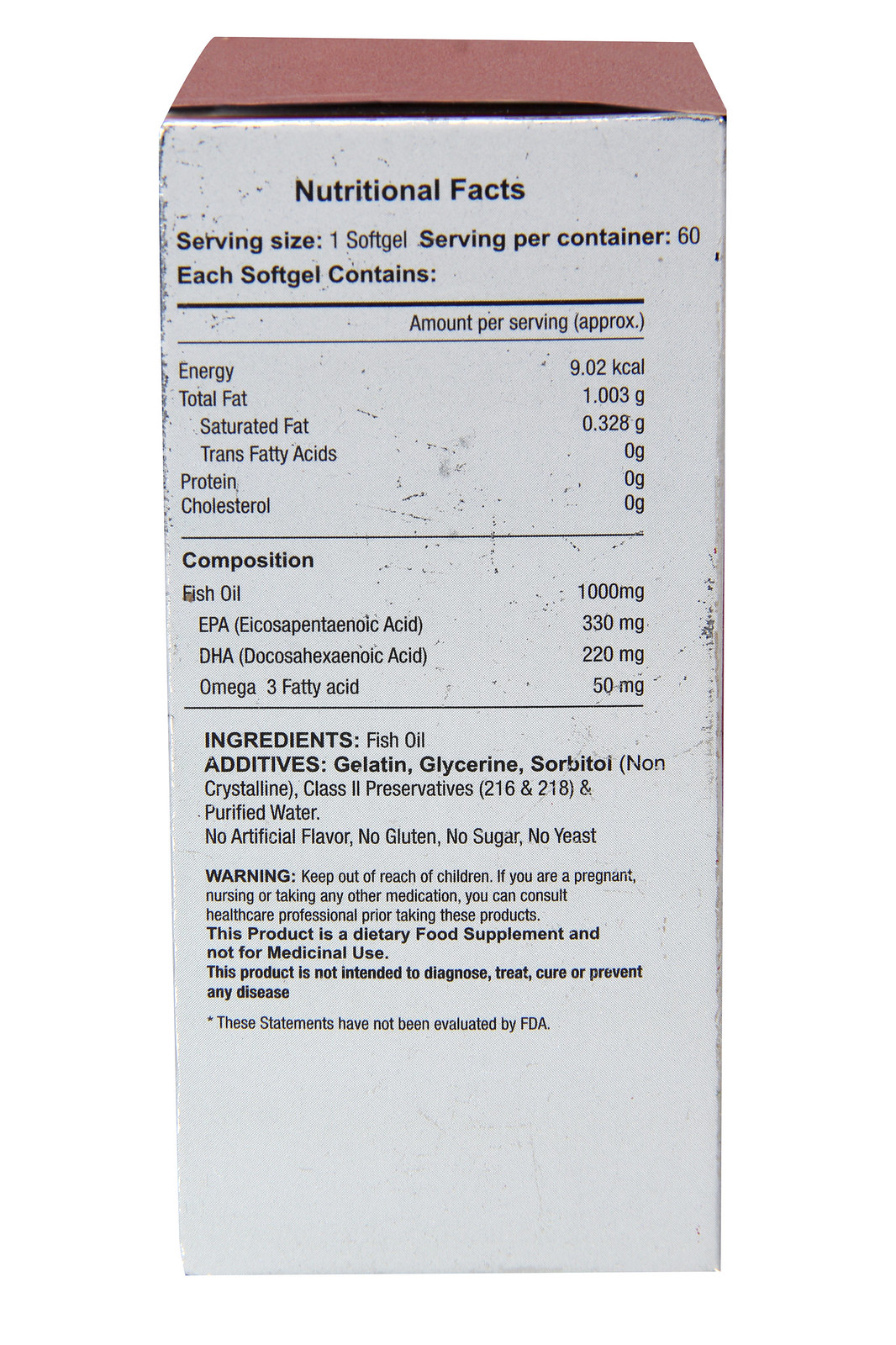The image shows the back of a dietary supplement box, featuring detailed nutritional information and additional product details. The top of the cardboard box is a purplish beige color, while the back is white with black text. The section begins with "Nutritional Facts" and outlines the serving size as one soft gel, with 60 servings per container. Each soft gel provides approximately 9.02 kcal of energy. It contains 1.003 grams of total fat, including 0 grams of trans fatty acids and 0.328 grams of saturated fat. The content includes 0 grams of protein and cholesterol. The primary ingredient is fish oil, with 1,000 milligrams per serving. This includes 330 milligrams of EPA, 220 milligrams of DHA, and 50 milligrams of omega-3 fatty acids. 

The ingredients list specifies fish oil, gelatin, glycerin, sorbitol, non-crystalline class II preservatives, and purified water. The product contains no artificial flavors, gluten, sugar, or yeast. A warning advises keeping the product out of children's reach and consulting healthcare professionals if pregnant, nursing, or taking medications. This dietary supplement is not intended for medicinal use and does not diagnose, treat, cure, or prevent any disease. The FDA has not evaluated these statements.